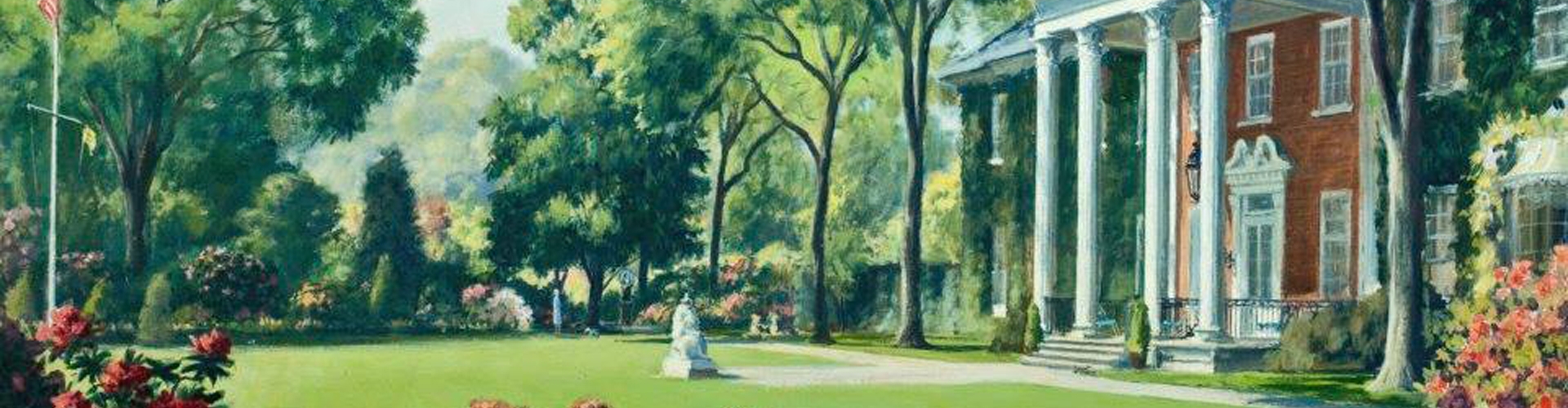The image is a detailed painting of a grand, older brick mansion, depicted in a long, vertically oriented frame. The house, which exudes the charm of a million-dollar home, features prominent white pillars and steps at the entrance. Accents of white trim around the doors and windows enhance its stately appearance. The building is partly covered with patches of moss or grass. 

In the foreground, a tidy walkway, flanked by a black gate, leads up to the white steps. The garden is brimming with vibrant flora, including clusters of yellow, red, pink, and white flowers, vividly scattered at the bottom right and left corners of the scene. A hint of greenery frames the base of the mansion, contributing further to the lush atmosphere.

Central to the composition, though somewhat obscured, is a statue that could possibly depict a lion. This statue is nestled amidst the greenery, serving as a striking focal point. The background reveals a dense cluster of tall, leafy trees, their green canopy stretching upwards and providing a serene setting. A flagpole can be faintly seen to the left of the house, against a backdrop of a clear blue sky, completing this picturesque scene.